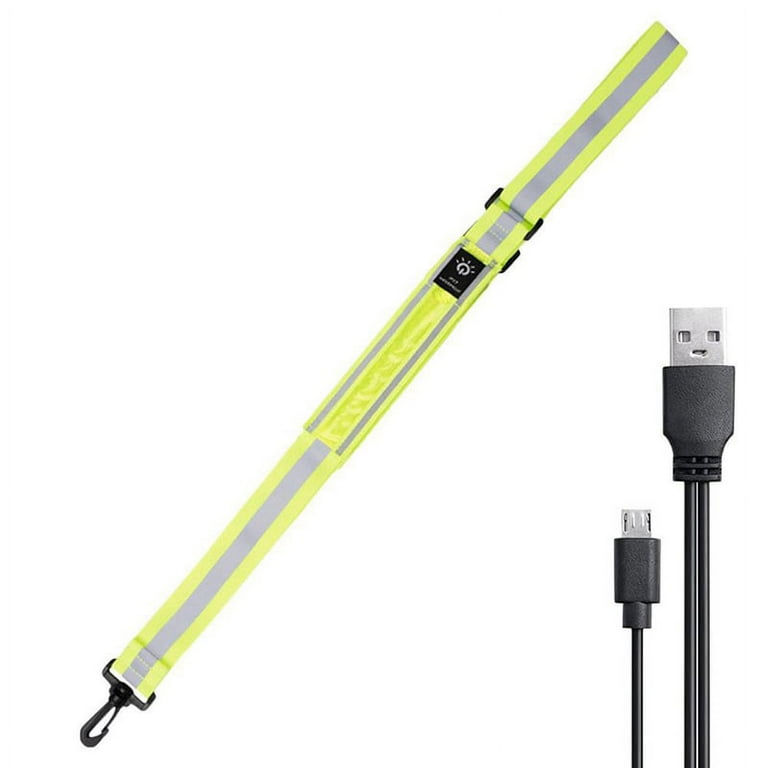The image presents a white background featuring a lime green and gray-striped strap running diagonally from the upper right to the bottom left. The strap, likely designed to secure devices, has a black clip at one end and a small black label. The lower right corner shows two black USB charging cords, one appearing to have a larger USB connector and a double cord configuration, while the other has a smaller connector with a single cord. The detailed view of this product, possibly for stock imagery, showcases both the strap and the accompanying charging cables, hinting at their use for electronics, such as phones or other devices.